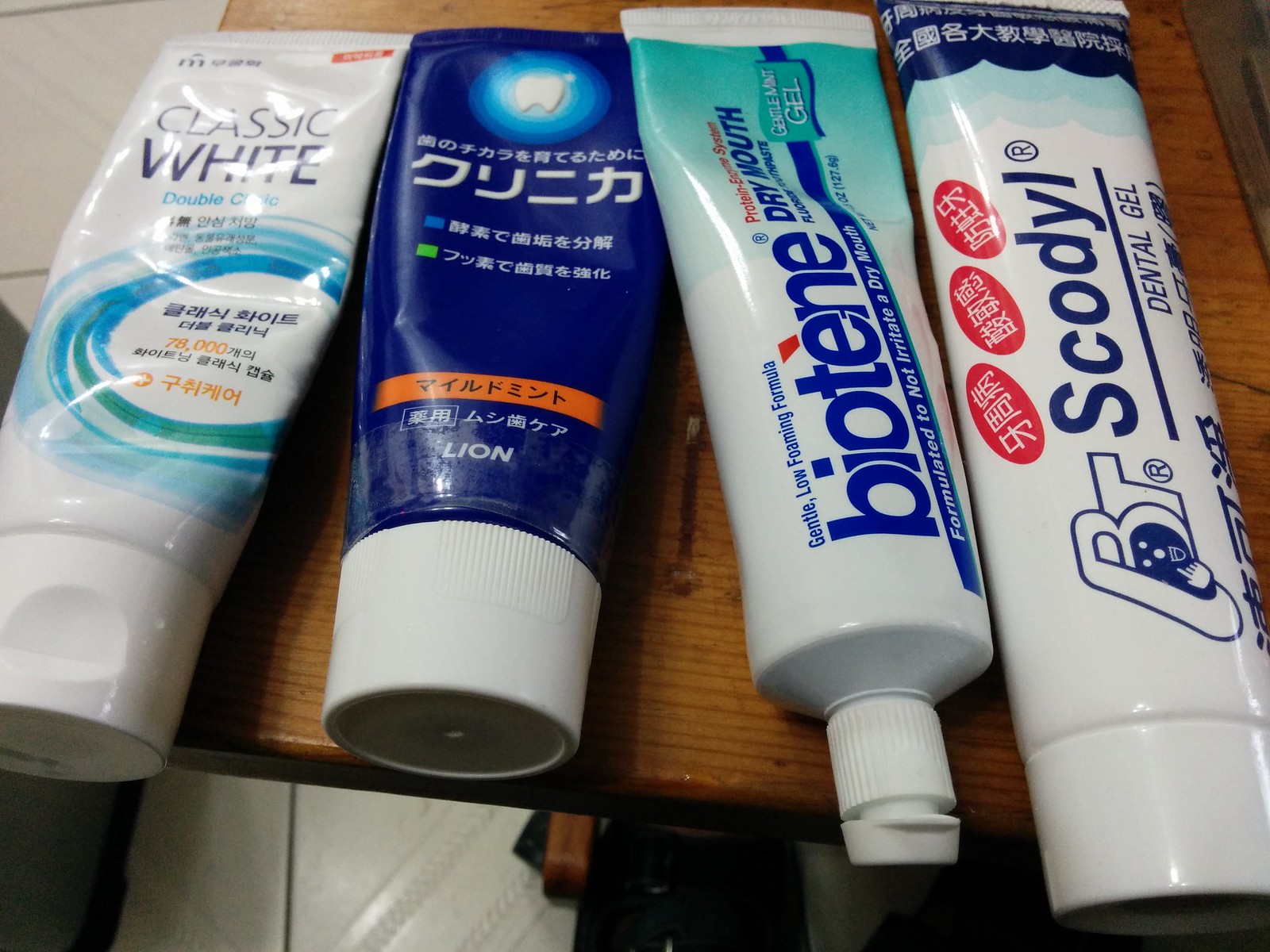The overhead close-up photo features four toothpaste tubes laid out in a neat row on an unpolished wooden table, perfectly aligned and slightly overlapping each other. The wooden surface, likely hardwood, showcases its natural lines, adding a rustic touch to the scene. 

From left to right: the first toothpaste tube is predominantly white with a "classic white" label and Korean script beneath, adorned with a swirl of blue and green. The second tube stands out with its dark blue color and Japanese writing, accompanied by an orange rectangle near the cap and the word "Lion" in English at the bottom. The third tube is white and labeled "biotene," with a tagline emphasizing "gentle low foaming formula formulated not to irritate a dry mouth," its cap slightly ajar. The final tube, also white, is marked "Scodial Dental Gel" with blue text and distinctive red slanted ovals above the name. Notably, this tube features a playful logo of a face within the bottom loop of the letter 'B,' smiling with a pointing finger. The table is set against a background of white tiles with streaked designs, hinting at a bathroom setting.